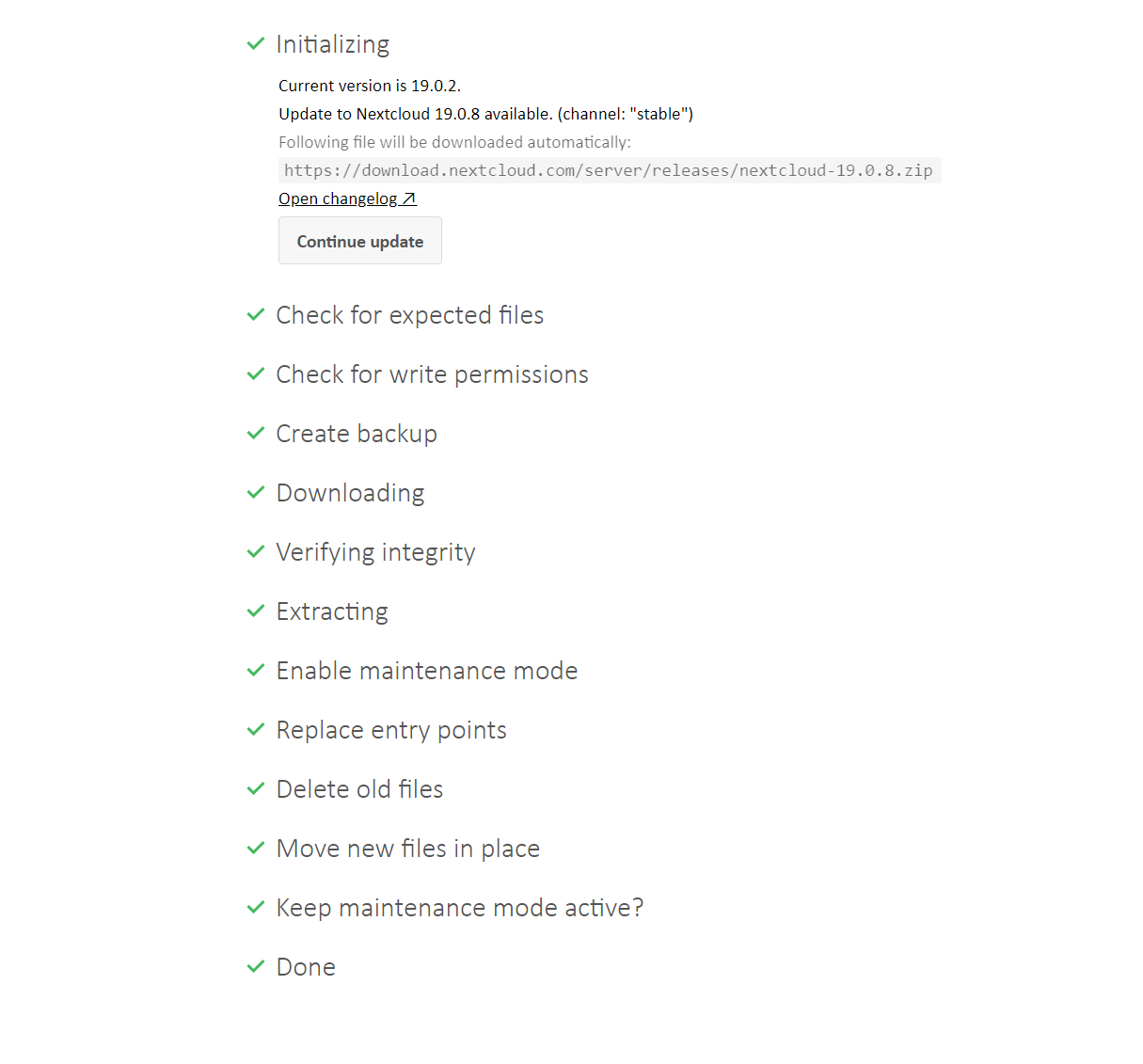The image displays a computer screen set against an all-white background, showcasing a software update interface for Nextcloud. At the top of the screen, the word "Initializing" is highlighted with a green checkmark next to it. Below this, in darker gray letters, the text reads, "Current version: 19.0.2." Further down, another text line indicates, "Update to Nextcloud 19.0.8 available", followed by a note in parentheses: "(channel: 'stable')".

Continuing down the screen, there's text indicating that a file will be downloaded automatically, followed by the address of a .zip file. Beneath this, a prompt to "Open changelog" is displayed. Moving further down, there is a small, outlined rectangle containing the text "Continue Update."

Underneath "Continue Update," there is a list of update steps, each accompanied by a green checkmark. These steps include checking for expected files, verifying write permissions, creating a backup, downloading, verifying integrity, extracting files, enabling maintenance mode, replacing entry points, deleting old files, moving new files into place, with a final checkbox stating, "Keep maintenance mode active?" The last item is marked "Done."